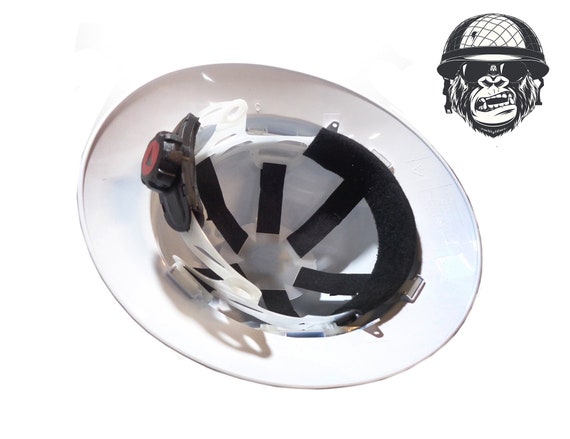This image captures an upside-down, white or silver plastic helmet, revealing its cushioned interior designed for head protection. The interior features several straps and velcro for securing the head, and a dial mechanism on the side for adjusting the fit. The helmet's visible section suggests it is sturdily built, likely for construction or industrial use. In the top right corner of the image is a logo depicting a menacing gorilla wearing sunglasses and a military-style helmet with a web or netting pattern, akin to a Vietnam-era helmet. This logo likely represents the helmet's brand, emphasizing strength and durability.